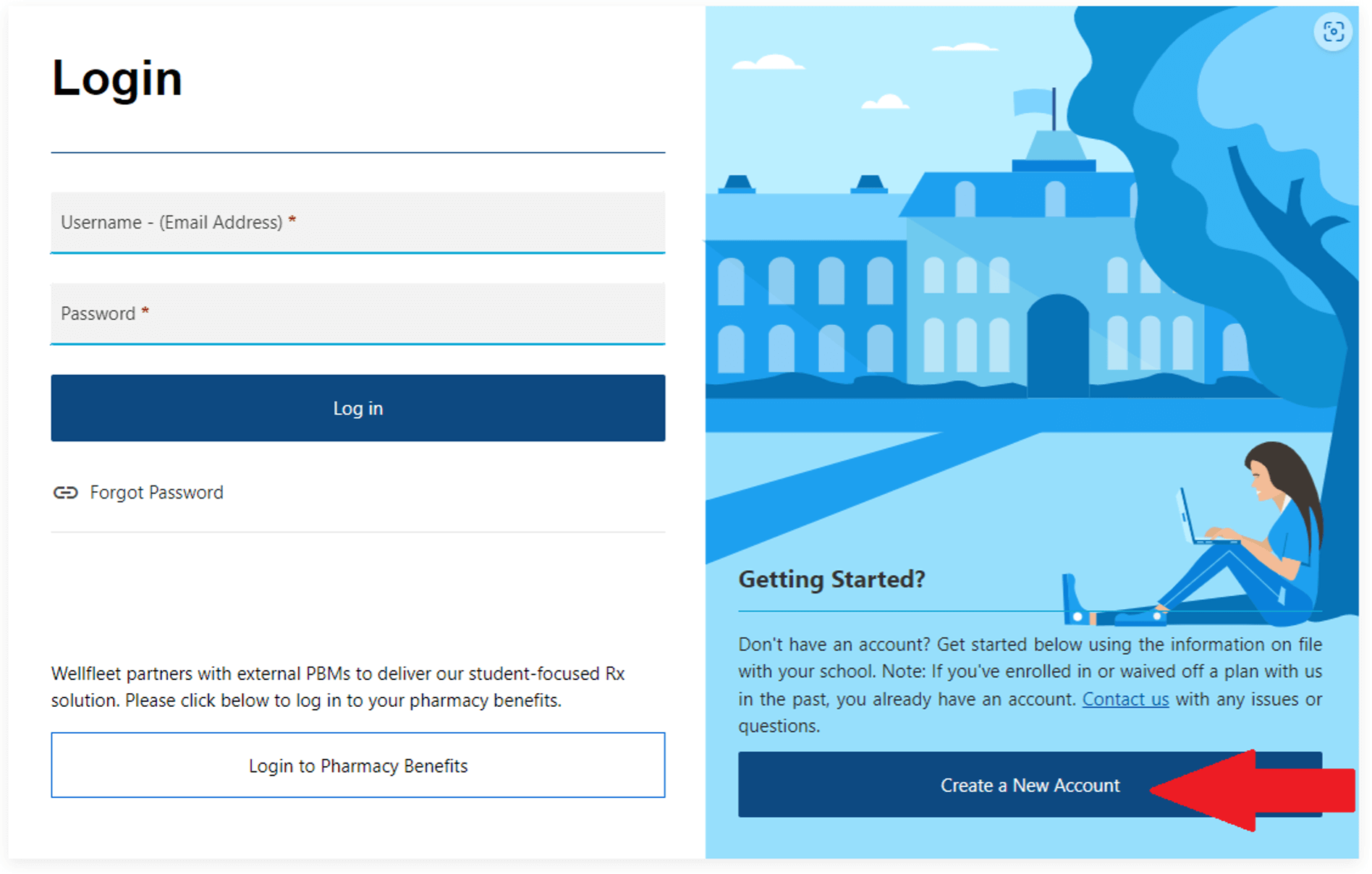**Image Description: Comprehensive Login Page for Student Services**

On the left side of the image, there is a white login box with a header titled "Login" at the top. Below the header, there is a horizontal line separating it from the rest of the content. Underneath the line, the following elements are arranged sequentially:

1. **Username Field**: A text box labeled “Username, email address” prompting the user to enter their credentials.
2. **Password Field**: Below the username field, another text box labeled “Password” for password entry.
3. **Login Button**: A blue button labeled “Login” for submitting the credentials.
4. **Forgot Password Link**: Under the login button, there is a link labeled “Forgot password” for users to recover their login information.

Further down the page, a segment reads: "Wellfleet partners with external PBMs to deliver our student-focused RX solution. Please click below to login to your pharmacy benefits." Beneath this statement is a large rectangular white button labeled “Login to pharmacy benefits.”

On the right side of the image, there is an artistic illustration featuring a blue-toned, multi-story building with a flag on its roof. In the foreground of the illustration is a woman sitting under a tree with her back against it, working on a laptop. Adjacent to this graphic, the text reads: “Getting started? Don’t have an account? Get started below using the information on file with your school. Note: If you’ve enrolled in or waived off a plan with us in the past, you already have an account.”

This comprehensive layout offers users clear instructions and access points for logging in and managing their accounts, emphasizing both student and pharmacy benefits.